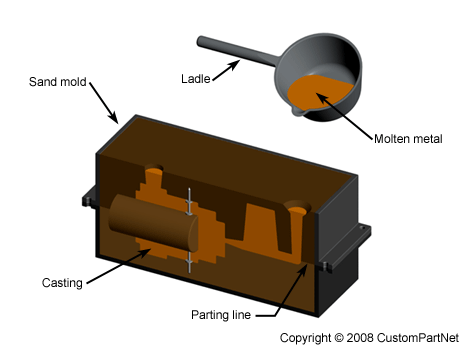This image features a detailed, cartoon-style diagram illustrating a casting process. At the top, there is a labeled ladle, depicted in gray and containing orange molten metal, with arrows indicating its contents. Below the ladle, a rectangular, brown sand mold is prominently displayed. The mold itself contains various shapes and design elements that suggest it has been prepared to receive the molten metal. On the left-hand side of the mold, an arrow points to the label "sand mold," while another arrow identifies a "casting" within the mold. Additionally, an arrow on the right-hand side points to a "parting line" that differentiates the dark brown and light brown sections within the mold. The entire illustration is set against a white background, and the bottom right-hand corner features a copyright notice: "© 2008 custompart.net." Overall, the image serves as an educational depiction of the casting process.